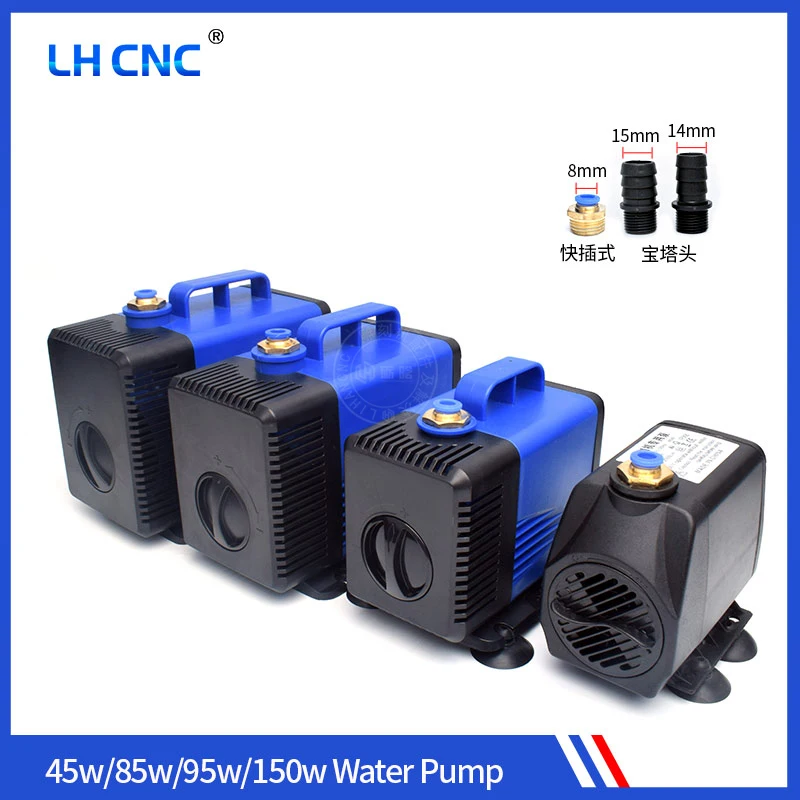This image is an advertisement for LHCNC water pumps, showcasing four distinct models arranged from largest to smallest from left to right. The three largest pumps feature a blue body with a black front and a handle on top, while the smallest pump, on the far right, is entirely black. Each pump has an outlet on top equipped with pipe threads. The power specifications—45W, 85W, 95W, and 150W—are displayed in white text on a blue background near the bottom, accompanied by a slanted graphic pattern of white, blue, and red bars, possibly incorporating the brand's logo. Additional fittings are shown in the upper right corner, including a brass-threaded fitting and another likely designed for hose press-fit connections. The text "LHCNC®" appears in the upper right, alongside some Asian characters beneath the fittings. The pumps also feature suction cup bases for secure placement during operation.